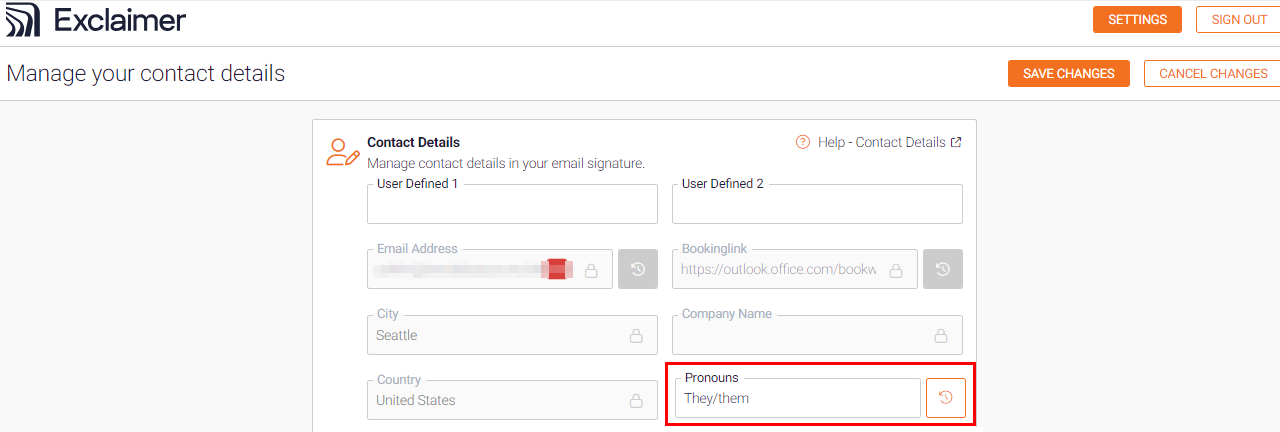This is a detailed screenshot of a website interface identified as "Exclaimer," with its name prominently displayed in black letters in the upper left corner. On the upper right corner, there's an orange "Settings" button with white text and a white "Sign Out" button with orange text. Below these buttons, the screen is split into two sections. The left section features the heading "Manage your contact details," while to the right, there are orange "Save Changes" and white "Cancel Changes" buttons.

Centrally located on the page is a primary box labeled "Contact Details" at the top left, with the "Help" option nearby. Immediately beneath this, there's a secondary heading: "Manage contact details in your email signature." Within this section, there are multiple input fields. The first two adjacent boxes are labeled "User Undefined One" and "User Undefined Two." Below these, there is a field labeled "Email Address" with an adjacent box labeled "Booking Link" containing the URL "https://outlook.office.com/book."

Further down, there are fields designated for "City" with "Seattle" entered, and "Company Name." At the very bottom of the page, two additional fields are present: one labeled "Country" with "United States" entered, and another labeled "Pronouns" displaying "they/them."